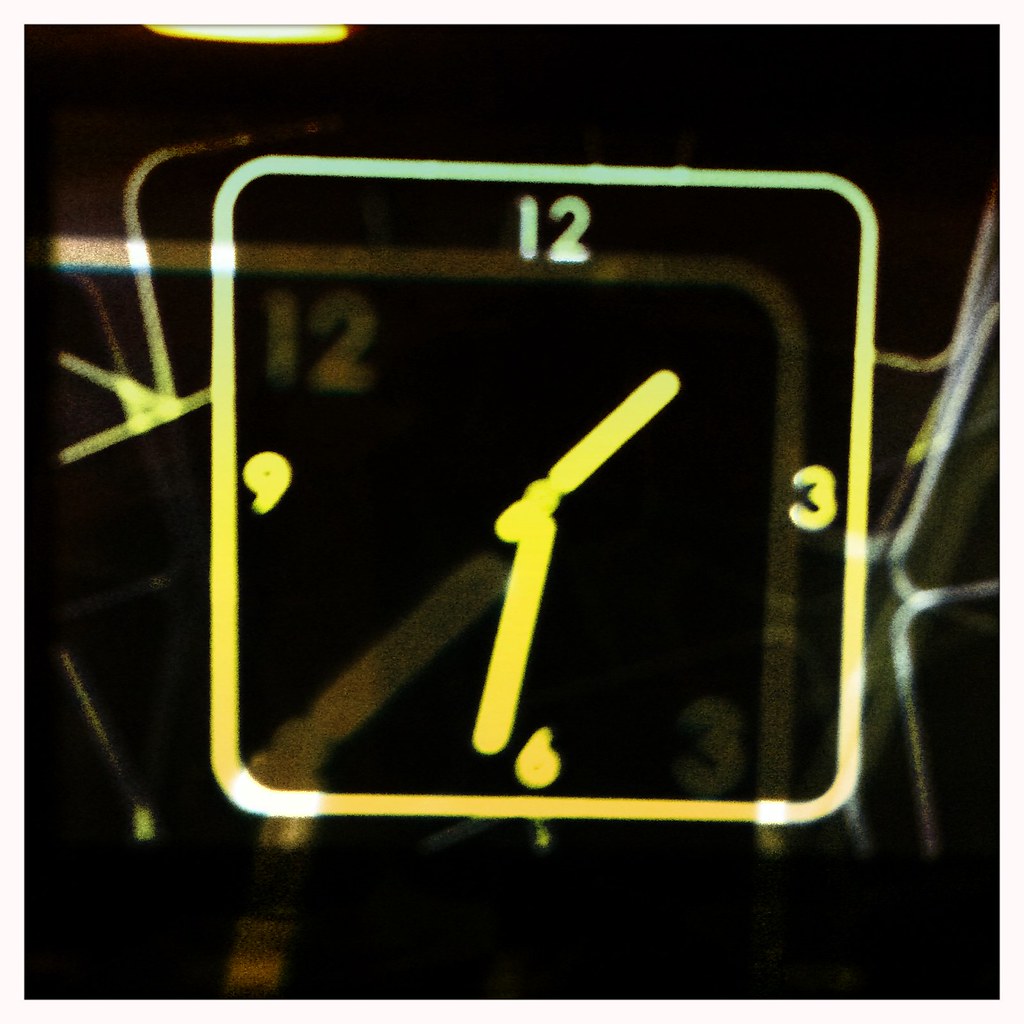The image depicts a clock with a unique, black, reflective surface, creating an almost double-image effect where the clock appears with a shadow-like reflection. The clock face is illuminated with neon lights at the cardinal points (12, 3, 6, and 9), each glowing vividly. The neon line at 12 o’clock is entirely green. Moving clockwise, the line from 3 o’clock transitions from green to yellow to a super light orange. The line from 6 o’clock shifts from light orange to a deeper orange. Finally, the line from 9 o’clock gradates from deep orange to yellow and back to green, completing the sequence. This vibrant array creates an engaging and colorful visual against the sleek black backdrop, enhancing the ethereal reflective quality of the surface.